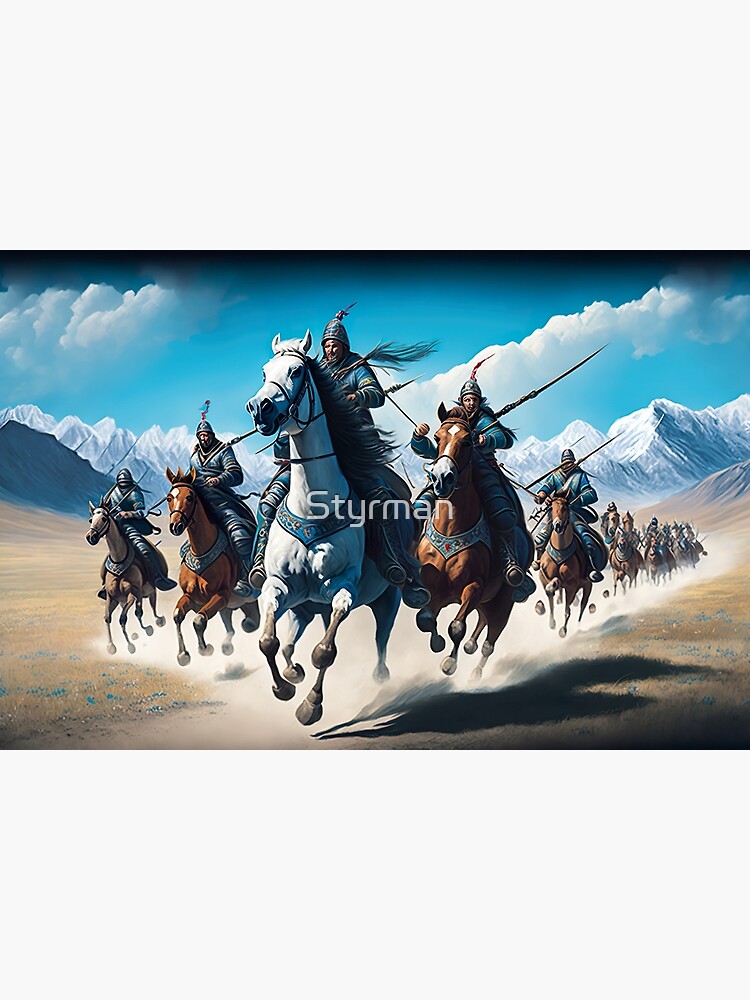This digitally animated artwork resembles a high-quality poster, depicting an action-packed battle scene inspired by the ancient Huns. Against a backdrop of a vivid blue sky accented by a dramatic, shadowy horizontal stripe, white clouds gather towards the bottom right. Central to the composition is a formidable mountain range stretching horizontally. Prominent in the foreground is a dynamic scene of warriors astride horses, charging forward on a dusty road. The formation is led by a distinguished warrior on a white horse, followed by a line of warriors on brown horses, creating a distinct V-shape. These animated characters are dressed in traditional Hun armor, complete with war helmets and spears pointed fiercely towards the right, evoking a sense of imminent conflict. This compelling imagery is completed with the detailed backdrop of glaciers, enhancing the scene's dramatic and historic feel.